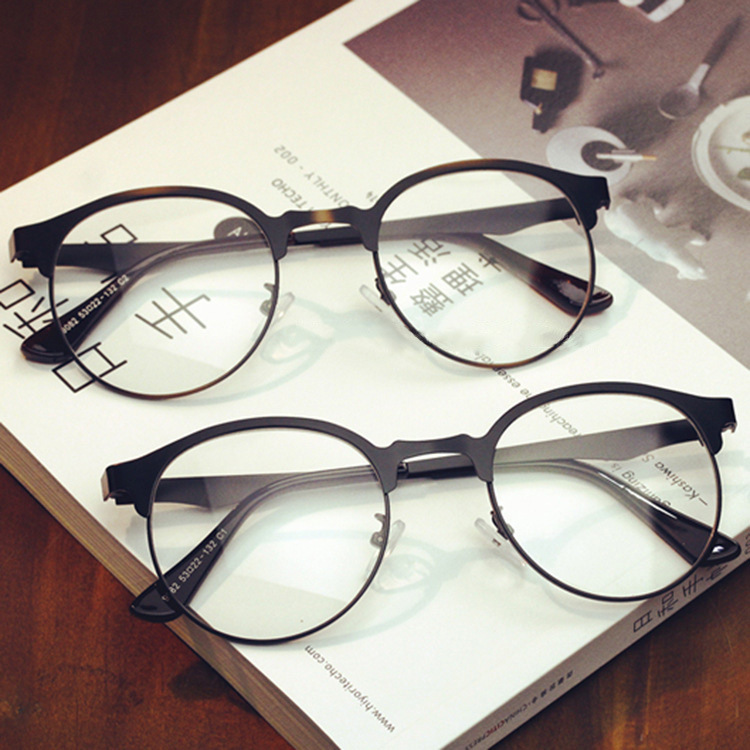The image shows two pairs of round eyeglasses resting on a magazine with a white cover that features Japanese text. One pair of glasses has a black frame, while the other pair features a tortoiseshell brown design. Both frames have an upper-only rim style, leaving the bottom part of the lenses exposed. The magazine, which is mostly in Japanese, also includes some English text like "Teco" and "monthly 002." The cover displays various design elements, including images of a polar bear, spoon, cigarette ashtray, jar, and scissors clustered in the upper right-hand corner. This setup is placed on a dark hardwood table. There are some letters and numbers on the armband of one of the glasses, though they are difficult to read, appearing as 8253022-132G1. The bind of the magazine, as well as the lower-right corner, also features some writing.